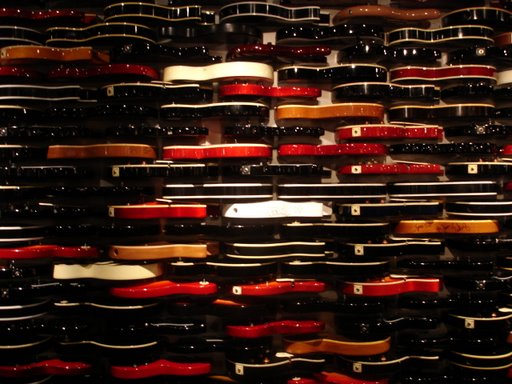This image portrays a display of multiple guitars of various colors, prominently arranged on a white wall within an indoor setting, potentially a store or museum. Most of the guitars share a uniform shape and thickness, though there are slight variations in their dimensions. The guitars are predominantly black, red, white, orange with white stripes, and shades of tan and brown. 

Some are particularly shiny, reflecting an artificial light source that is illuminating the display. This light creates varied intensities of brightness on the guitars, emphasizing their glossy finishes. The arrangement of the guitars appears horizontal, allowing the viewer to see their curved sides. 

The backdrop is a white wall, enhancing the contrast and visibility of the differently colored guitars. Overall, the display exudes a sense of artistic organization, highlighting the aesthetics and diversity of the guitars.